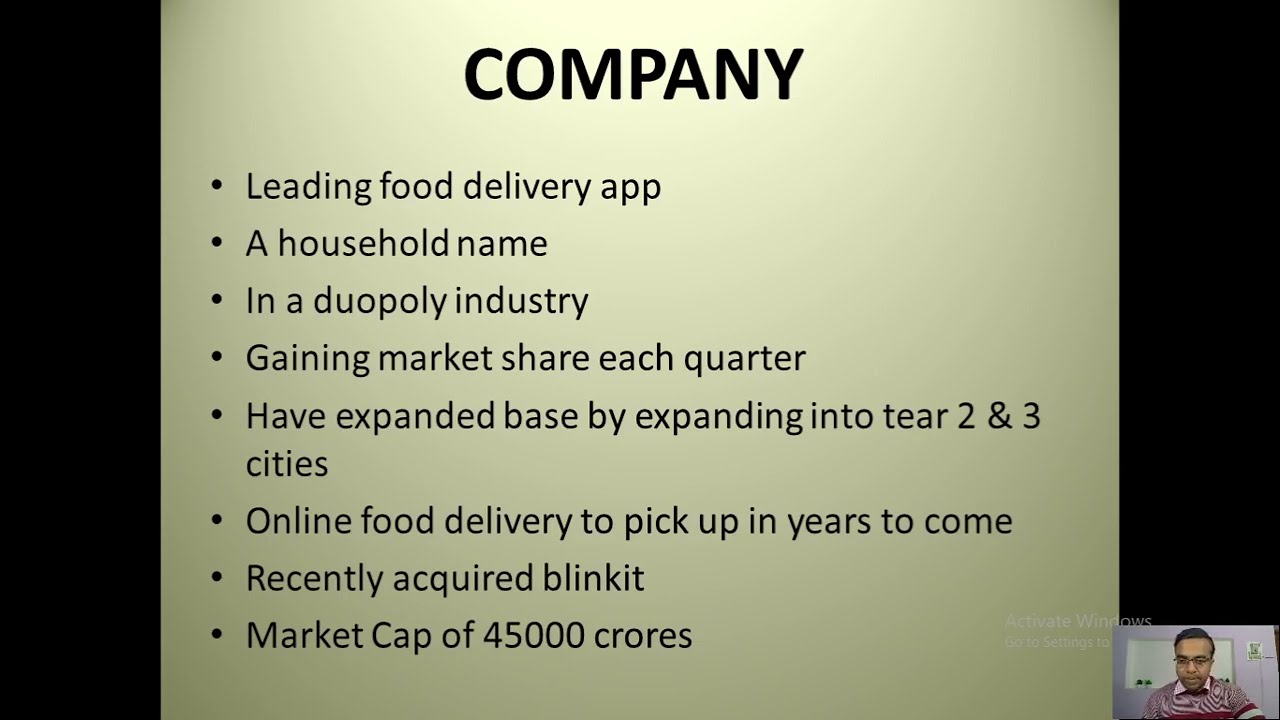The image is a screenshot from a presentation slide, framed on the left and right by vertical black rectangles. In the bottom right corner, there is a small video capture of a man who appears to be of Indian or African-American descent, wearing glasses and a red and white collared shirt. The majority of the slide's background is a light greenish-brown color. At the top center, the word "company" is prominently displayed in bold black print. Below, a series of bullet points outline key details: "leading food delivery app," "a household name," "in a duopoly industry," "gaining market share each quarter," "expanded base by expanding into tier two and three cities," "online food delivery to pick up in years to come," "recently acquired Blinkit," and "market cap of 45,000 crores (C-R-O-R-E-S)." Additionally, there is a visible watermark at the bottom that reads "activate windows, go to settings." The colors present in the image include black, light green, purple, red, orange, tan, and gray.